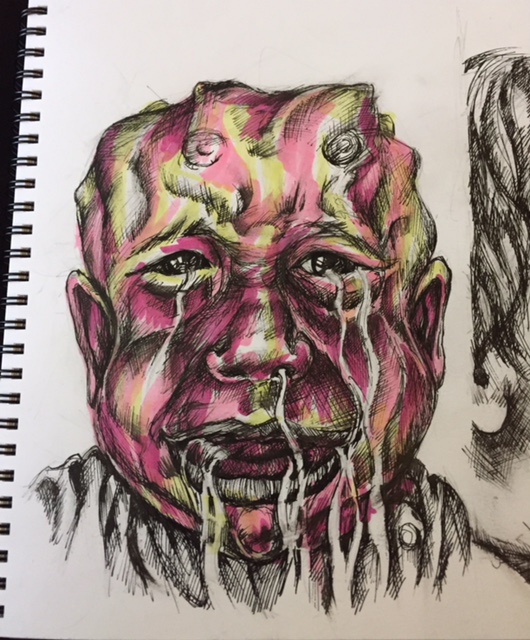The image features a vibrant and detailed drawing, characterized by its bright yellowish-green, pink, and purple hues, set against a stark white background of notebook paper. The paper is part of a notebook bound by black metal rings, visibly punctured through the left margin. 

To the right edge of the paper, there is an additional partially visible sketch rendered in pen or pencil. Its lines appear scratchy and indistinct, making it hard to discern the subject of this secondary drawing.

The main focus of the artwork is a striking, almost humanoid face that appears mutated. The head is hairless and not perfectly round, with textured ridges and contoured edges. Its ears lie flat against the sides of the head, adding to the unusual appearance. The face features exaggerated facial elements, including large lips and a prominent nose. It is predominantly painted in shades of red or pink, with a vivid lime green stripe running down its face, sparing the areas around the eyes, which are depicted in a stark black.

Emphasizing the emotive quality of the piece, a single tear falls from the left eye, paralleled by two tears streaming from the right eye. Additionally, there is liquid trickling from the nose and mouth, enhancing the sense of distress or mutation conveyed by the artwork.